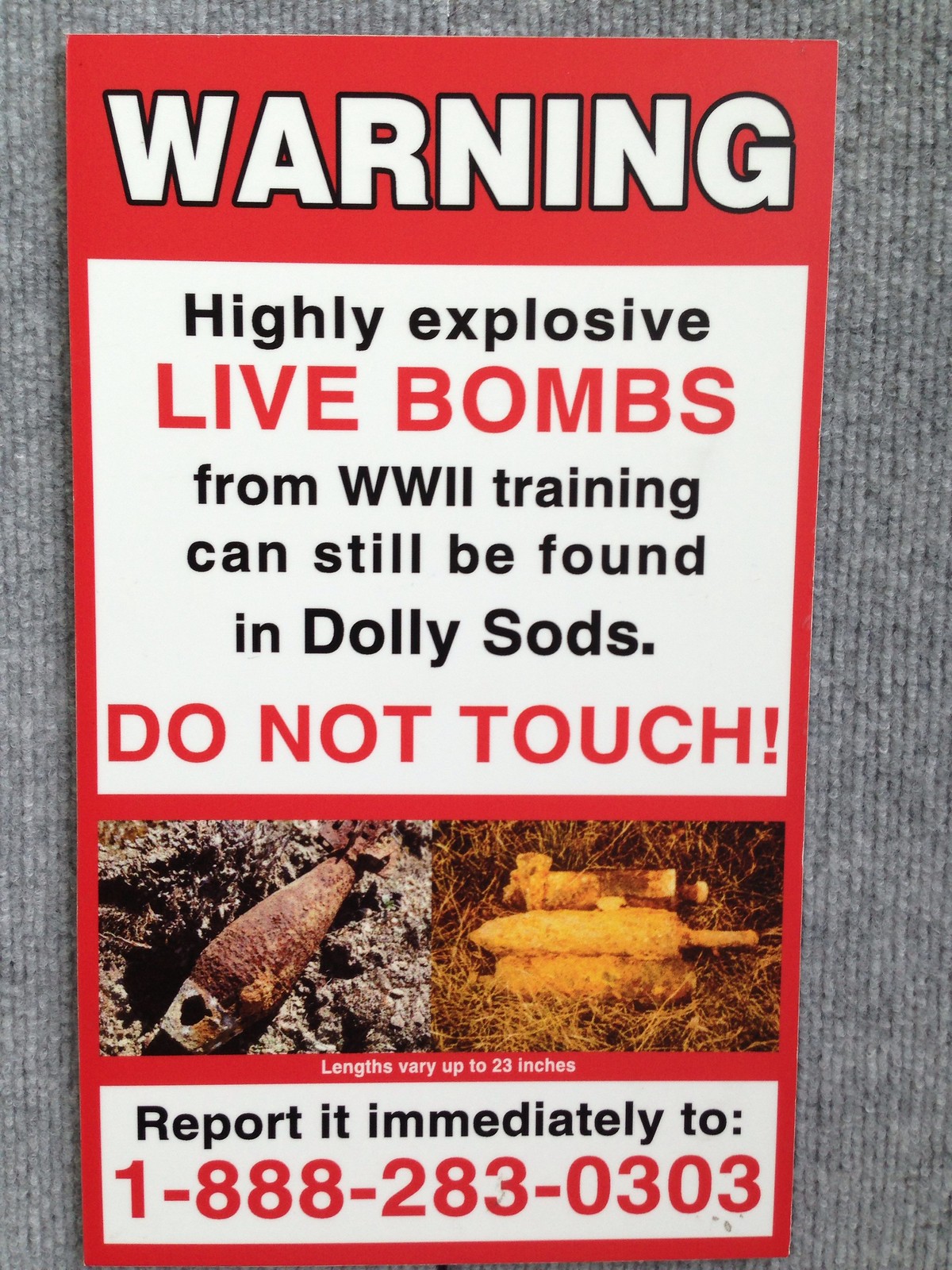The image displays a warning sign on a gray carpet. The sign is vertically oriented with a prominent red background and borders. At the top, in large white capital letters outlined in black, it reads "WARNING." Below this, a central white square contains the following message in various colors: "HIGHLY EXPLOSIVE" in black, "LIVE BOMBS" in red, "FROM WW2 TRAINING can still be found in Dolly Sods" in black, and "DO NOT TOUCH!" in red. Beneath the text, there are two photographs on either side. The left photo depicts a rusted, squash-shaped metal item with a hole at the bottom, while the right photo shows three yellow, corn-shaped objects. The text beneath the images states, "LENGTHS VARY UP TO 23 INCHES" in white. At the very bottom, another white box contains the text "REPORT IT IMMEDIATELY TO" in black, followed by the phone number "1-888-283-0303" in red.